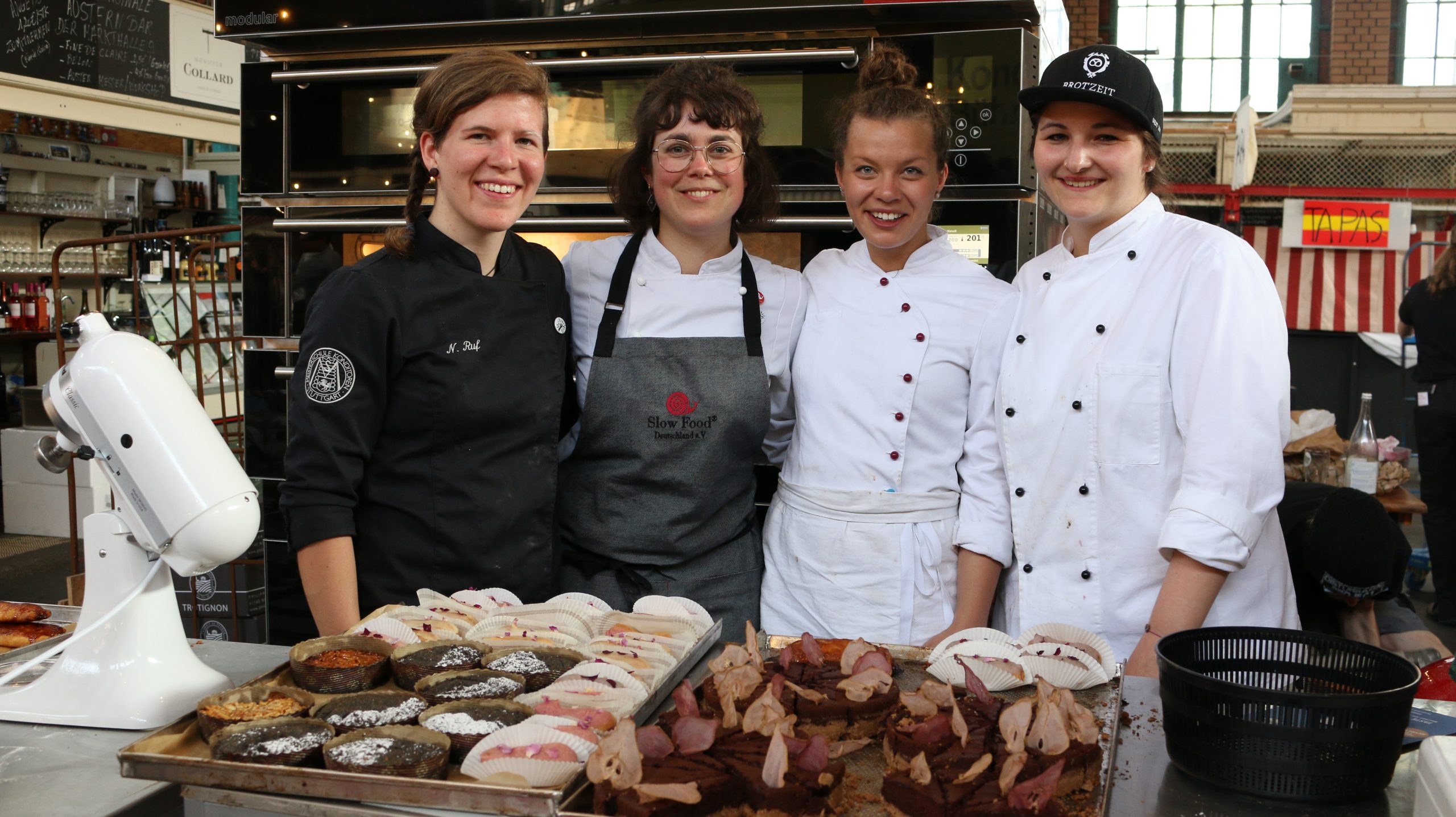The image features four joyful chefs, each adorned in distinct chef's attire; two are wearing crisp white jackets, one sports a white jacket with a black apron, and another is donned in a sleek black jacket. All four are Caucasian females, smiling broadly, exuding an air of camaraderie and excitement. In front of them lies an enticing array of culinary creations, including assorted desserts like brownies dusted with powdered sugar, miniature pie tarts, and various cookies and sliced barbecue meats elegantly displayed on trays. The table also features a white mixer, indicative of a professional setting, with an oven visible in the background, hinting that this scene might be from a cooking show or competition.